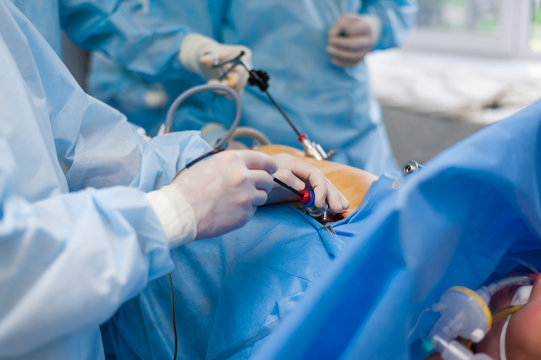The image depicts a meticulous scene within a brightly lit operating room. At the center lies a patient, partially covered by a blue surgical drape, with tubes meticulously placed around their face, indicating they are intubated. In the foreground, a doctor donned in light blue scrubs is actively engaged in a surgical procedure, wielding an unidentified tool against the patient's body, potentially administering an injection or utilizing a surgical instrument. Another medical professional, clad in darker blue scrubs, stands attentively in the background, possibly observing or assisting. Both practitioners are equipped with white latex gloves, highlighting the sterile environment. The clarity of the image is noteworthy, capturing every detail, from the texture of the surgical attire to the natural light filtering through what appears to be a window with a white frame in the background. The overall composition exudes a sense of precision and urgency characteristic of a live surgical setting.